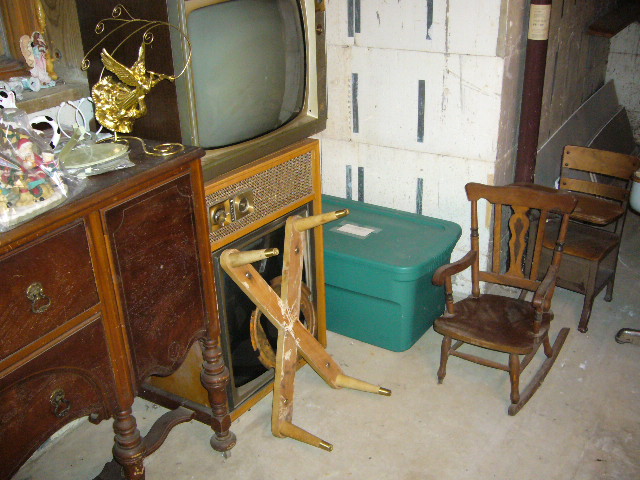The photograph depicts a cluttered storage area, possibly a basement or attic, filled with an assortment of vintage and antique items. Central to the image is a tube TV from the 1960s perched atop an old speaker with a potentially ripped speaker cover and a mounted hook in the shape of an X. Below and to the left, there is an intricately carved cherry wood console with dusty pull-out drawers, adorned with a gold angel decoration blowing a horn. Next to this is a dark wooden piece of furniture with missing handles and ornate carvings. Scattered around the unfinished, wood or concrete floor are a tiny child’s wooden rocking chair and an equally small, aged school desk, hinting at the presence of young children in the past. A steel beam cuts through the image, further emphasizing the unfinished aspect of the room, which is also cluttered with grey metal boxes, and a pile of storage boxes stacking haphazardly over each other. Exposed pipes in the ceiling and the general dusty ambiance contribute to the sense of neglected yet nostalgic storage space.